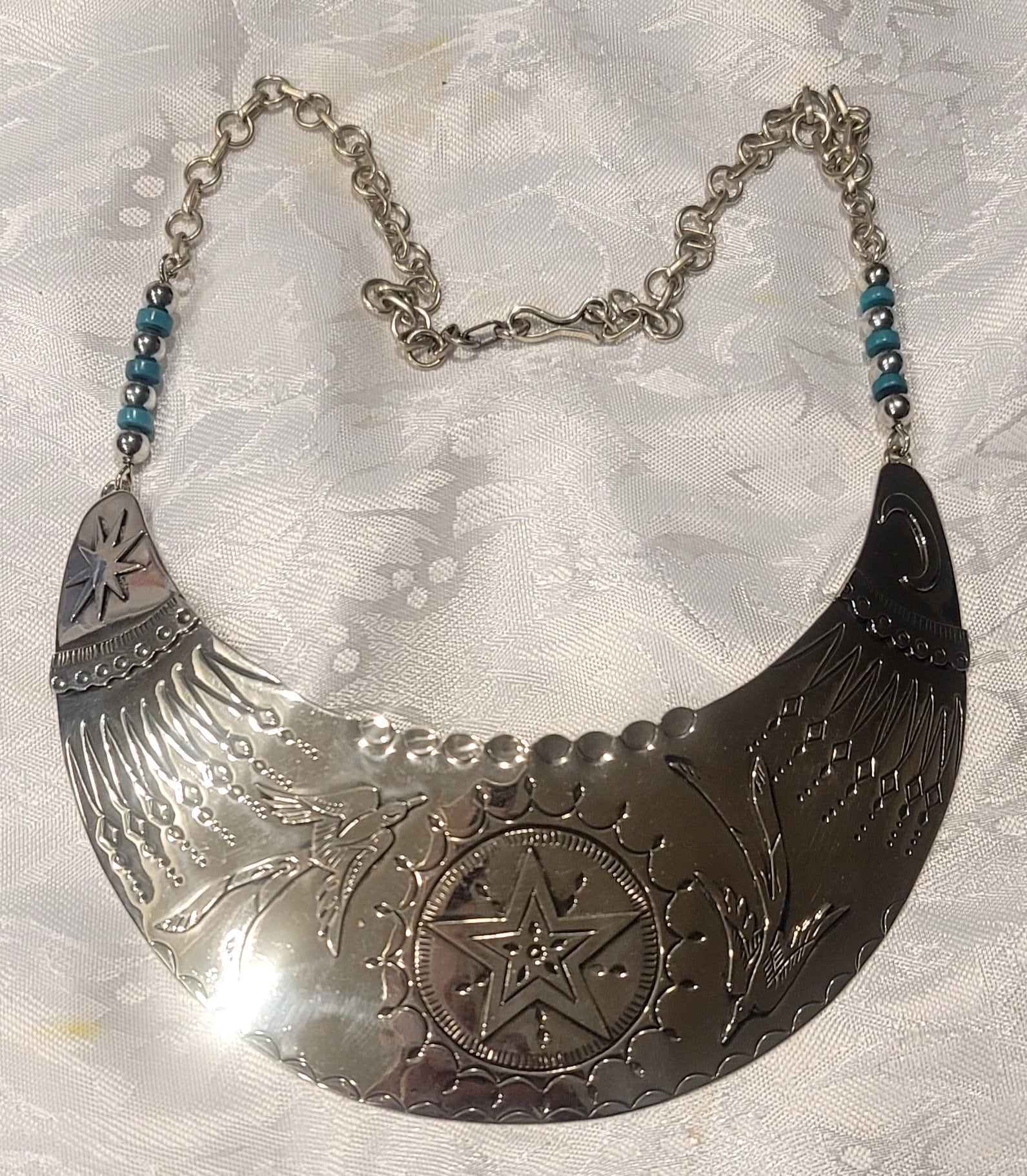The image features a large and intricate piece of jewelry, likely a necklace, designed with a chain of intertwined silver circles that encircles the neck. Suspended from this chain is a crescent-shaped pendant, crafted from a darker metal, possibly gray or bronze. The pendant exhibits exquisite detailing, including a meticulously chiseled bird on the left side and a flower on the right. Additionally, engravings of stars and other motifs, such as zigzag-patterned metal, adorn the half-moon shape. The center of the pendant prominently displays a star, resembling a sheriff's badge, set within a circle. Interspersed along the chain are green beads, organized in groups of three and intertwined with the metal links on both sides. The entire ensemble rests against a backdrop of gray and white fabric, highlighting its elaborate design and craftsmanship.